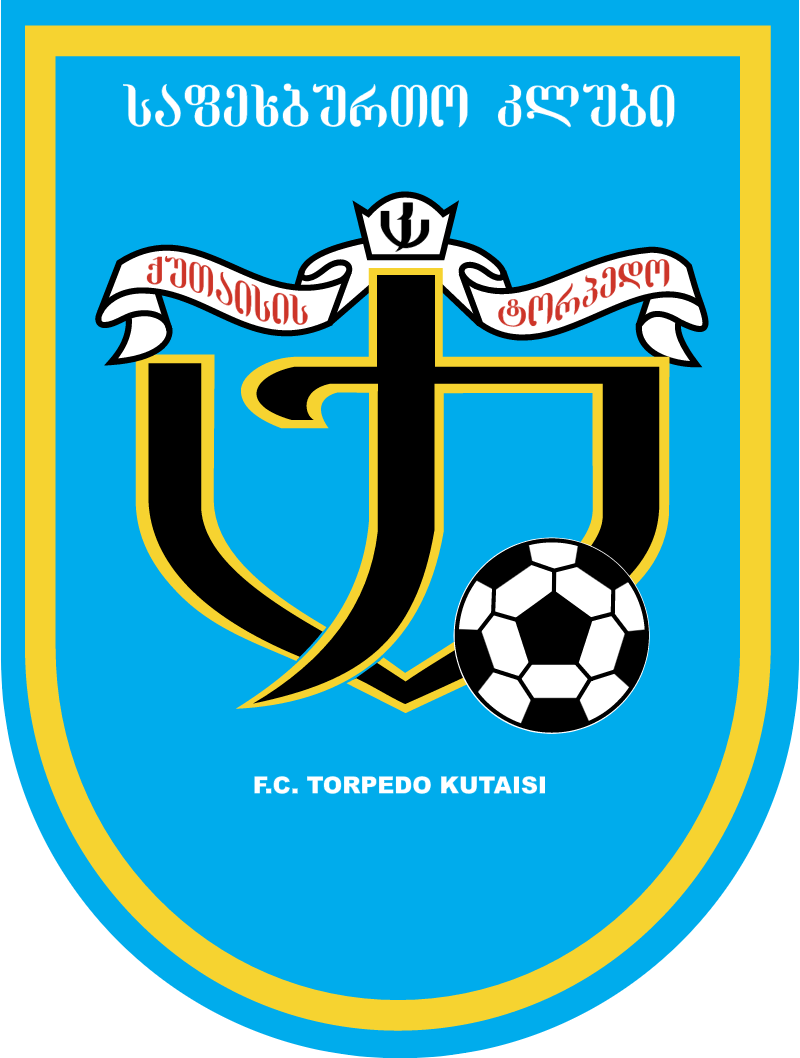The image showcases a flag or pennant for a soccer team, predominantly featuring a bright baby blue background with a yellow-orange border in a shield shape. At the top of the shield is white text in a foreign language, which appears unreadable. Just below this text is a white ribbon with red text, further contributing to the unique and intricate design. Central to the image is an insignia formed by the letter 'J' with a line extending and bending into a V-shape, culminating in an arch above the 'J'. This insignia is crowned with a crown shape from which ribbons drape to either side. A black and white soccer ball is positioned to the bottom right of the insignia. At the base of the image, white text reads: "F.C. Torpedo Kutaisi."